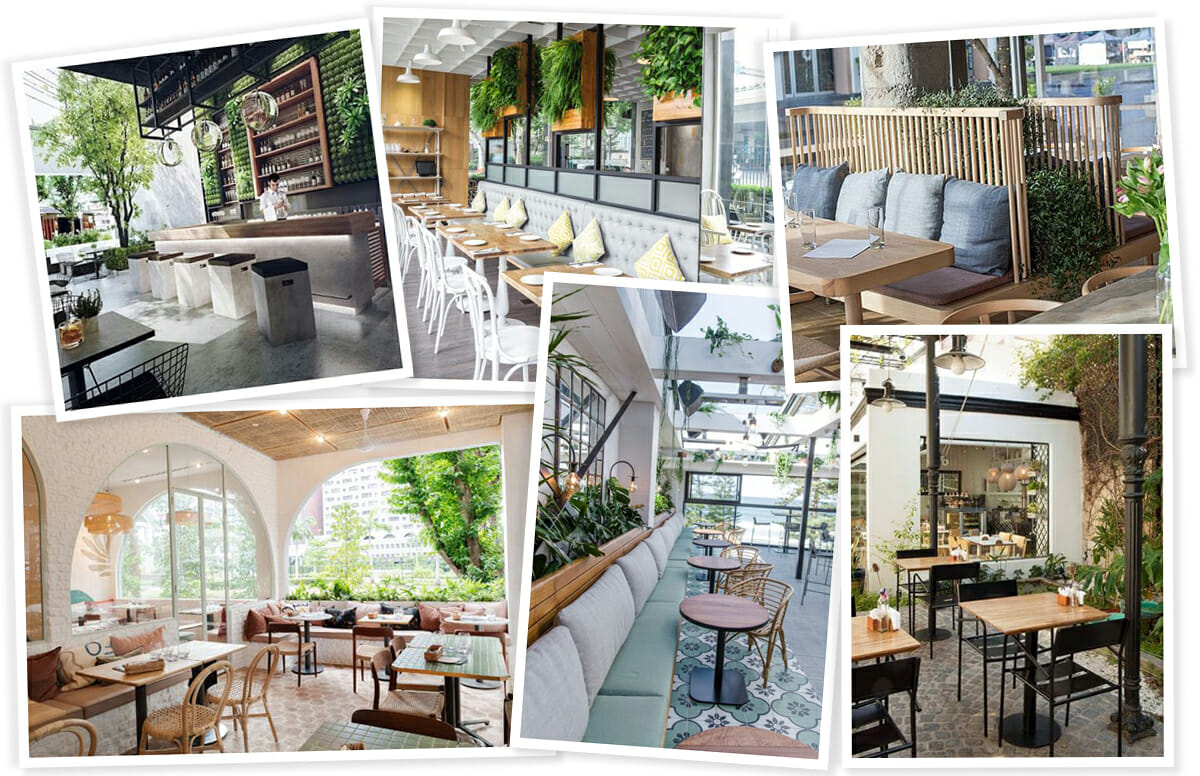This detailed collage features six white-framed 8x10 photographs, each capturing various aesthetically pleasing, open-air restaurant settings, highlighting diverse seating arrangements and design styles. 

The top-left image showcases a modern, open-air bar area with grey, modern furnishings, white square barstools, industrial black shelving, and lush greenery, exuding a chic, contemporary vibe. The upper-middle photo depicts a restaurant space featuring a large, cushioned bench with white chairs and wooden tables set against a backdrop of greenery and modern, grey-scale furniture, enhanced by a striking fern wall. The top-right picture offers a view of possible outdoor seating with extensive greenery, live plants, trees, latticework, and glassware on wooden tables, suggesting an airy, natural environment.

In the bottom-left corner, there's a sunny, well-lit dining area with large windows, square tables, and wicker chairs, framed by arched doorways and boasting a Mediterranean feel with a minimalist, brown and beige color scheme. The middle-bottom image reveals a Moroccan-inspired eatery featuring green tiled floors, wicker chairs, and potted green plants, complemented by grey furnishings and a modern aesthetic. Finally, the bottom-right picture highlights an alfresco Italian-style restaurant with black chairs, wooden tables, cobblestone flooring, and quaint old-fashioned streetlights interspersed among the lush greenery, completing the elegant collection with a touch of European charm.